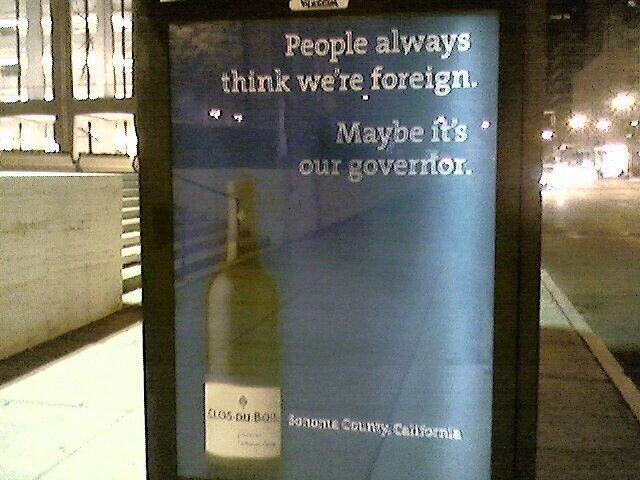The photograph captures a nighttime urban street scene featuring a bus stop enclosure on the sidewalk. The enclosure displays a brightly lit advertisement within a dark brown frame. The ad text reads, "People always think we're foreign. Maybe it's our governor," in white letters on a blue background, likely referring to the era when Arnold Schwarzenegger was governor of California. Below the text, a green bottle of Clos du Bois white wine from Sonoma County, California is prominently displayed with its label facing forward. The reflective surface of the ad suggests it might be glass. To the left, steps lead up to a large commercial building or a parking garage. In the background, city lights and car headlights illuminate the street, adding depth to the urban landscape.